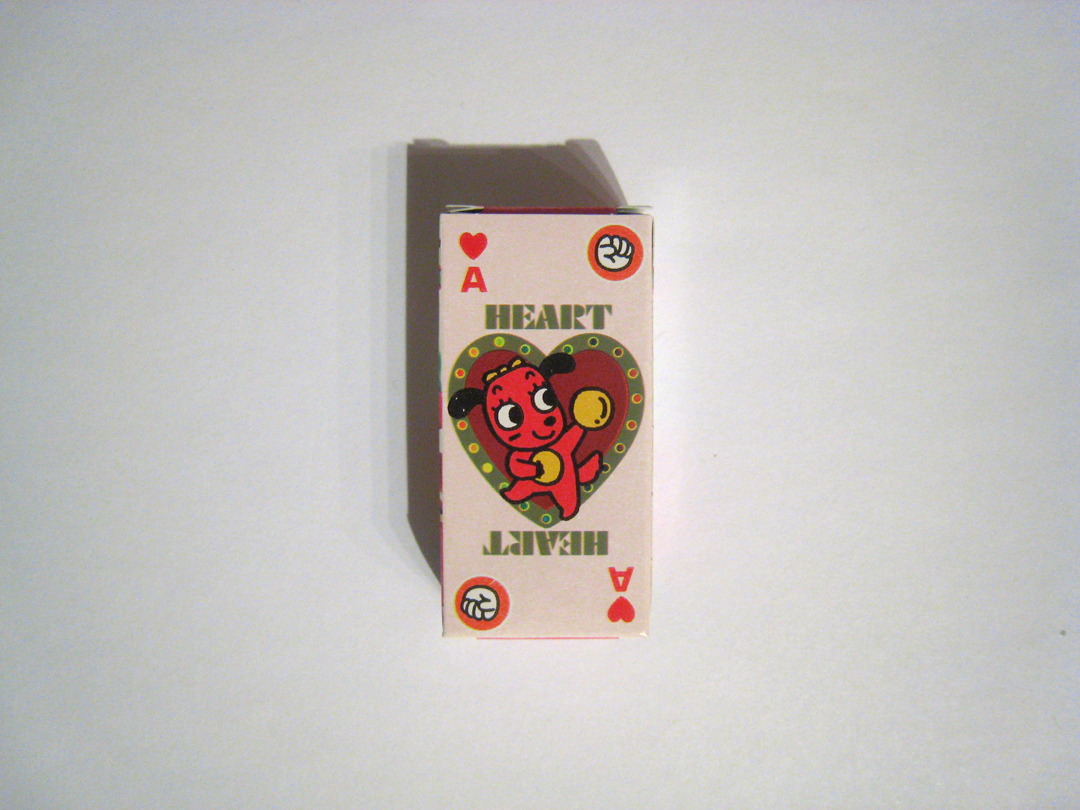This image features a rectangular box, photographed against a plain, light gray or white background, casting a subtle shadow towards the top left. The box is slightly elongated, diverging from the typical dimensions of a standard deck of cards, and is displayed in a portrait orientation. The primary background color of the box is a muted white.

Centrally positioned on the box is a large heart with a green outline filled with a myriad of colored dots resembling a confetti-like pattern. Inside this heart, there stands a small red dog with distinct black ears, black eyes, and holding two orange balls in its front paws. The dog also has a yellow bow on top of its head and stands upright on its hind legs against a reddish background.

Above this central heart, the word "HEART" is prominently displayed in green text, and below the heart, the same word "HEART" appears again but upside down. At the top left corner of the box, there is a red heart coupled with the letter "A," symbolizing the Ace of Hearts card. In the top right corner (and mirrored on the bottom), there is an orange circle containing a white fist. The same graphics—Ace of Hearts and fist in a circle—appear at the bottom two corners, but upside down.